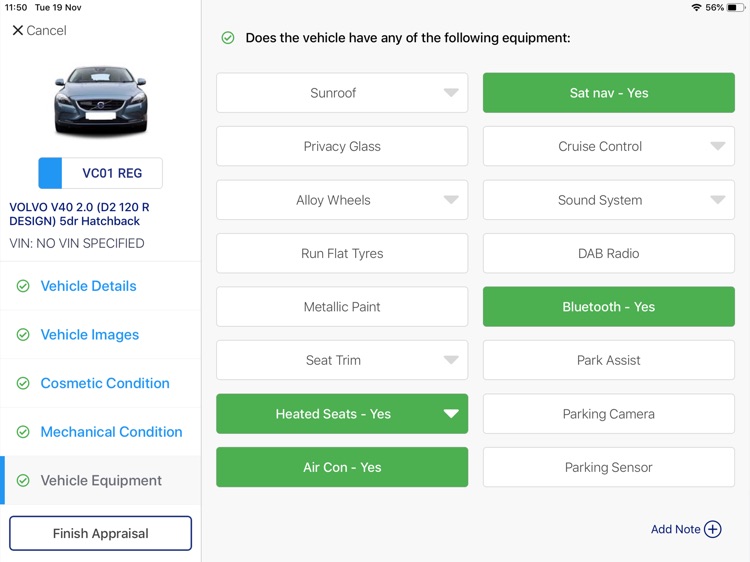**Descriptive Caption for the Image:**

The image features a detailed interface of a vehicle appraisal system. On the left, there is a vertical strip with a white background, displaying a sequence of information. At the top of this strip is a white bar with the text "1150 to 19" next to a clickable "X" labeled "Cancel".

Beneath this bar is an image of a car, specifically labeled as "Volvo V40 2.0 (D2 120 R-Design) 5dr Hatchback". Adjacent to the car, there's a button labeled "VCO 1 REG", which has a blue left side and a gray outline with blue font.

Below the car's information is a list of buttons including:
- Vehicle Details
- Vehicle Images
- Cosmetic Condition
- Mechanical Condition
- Vehicle Equipment

The "Vehicle Equipment" tab is currently highlighted. This section asks if the vehicle has certain features, with a series of dropdown menus and buttons indicating the presence or absence of each feature. The layout is as follows:
- Sunroof: (Dropdown menu)
- Privacy Glass
- Alloy Wheels: (Dropdown menu)
- Run Flat Tires
- Metallic Paint
- Seat Trim: (Dropdown menu)
- Heated Seats: "Yes" (Green button)
- Air Conditioning: "Yes" (Green button)
- Satellite Navigation: "Yes" (Green button)
- Cruise Control: (Dropdown menu)
- Sound System: (Dropdown menu)
- DAB Radio: (Dropdown menu)
- Bluetooth: "Yes"

At the bottom of the section, there's a button labeled "Finished Appraisal". The overall interface is designed to comprehensively detail the vehicle's features and condition.